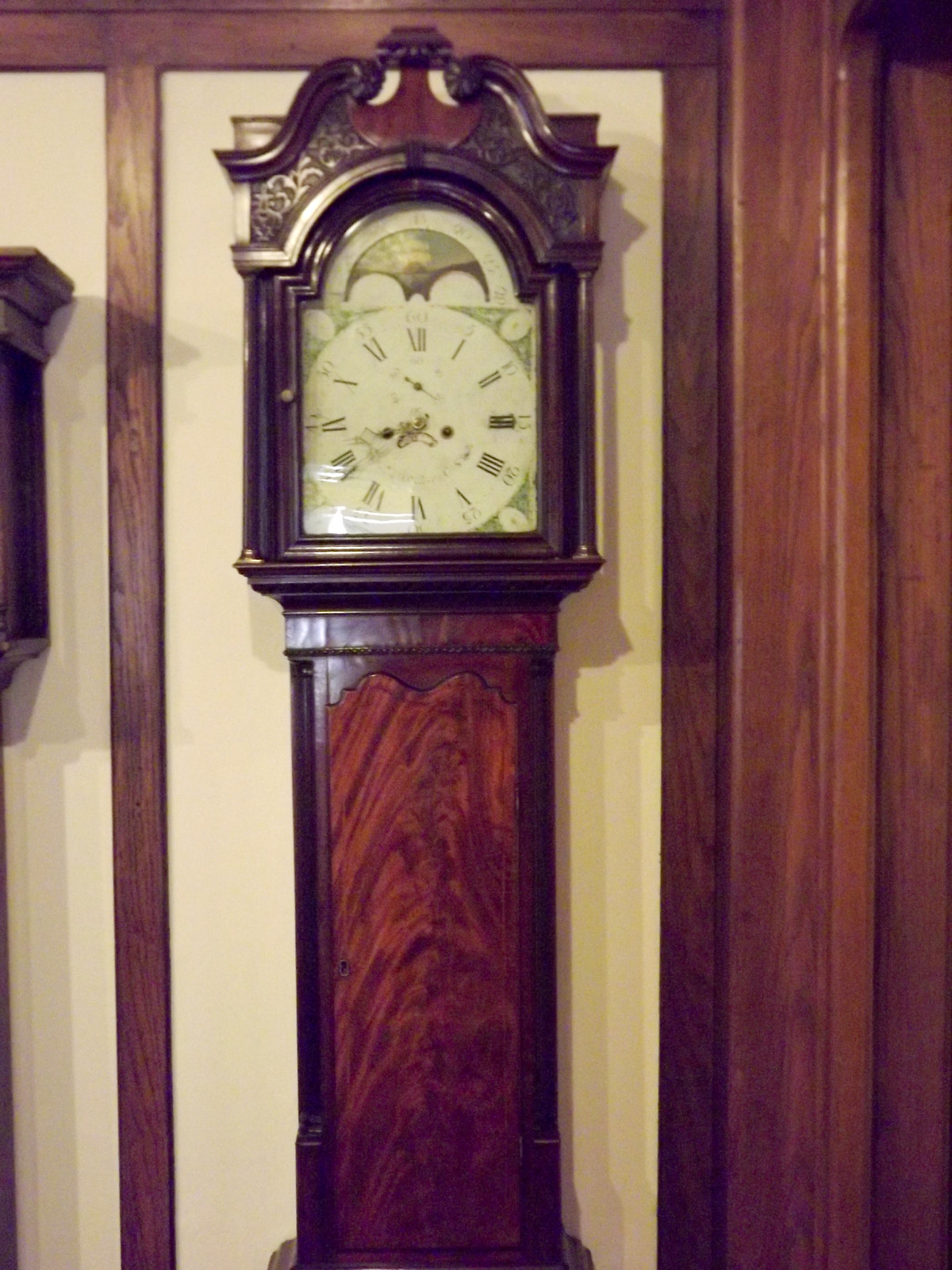In the image, a white-painted wooden wall serves as the backdrop, trimmed elegantly with rich brown wood. Centrally mounted is an elongated, vertically oriented, brown wooden plaque. At the top of this plaque rests an antique-style clock, featuring golden Roman numerals from 1 to 12. The time is indicated by matching golden hour and minute hands. To the left of this clock, another similar object is affixed to the wall, suggesting the presence of a second clock or possibly a decorative item. The overall setting exudes a rustic yet refined aesthetic, with the contrasting woods and gold elements providing a touch of classic elegance.